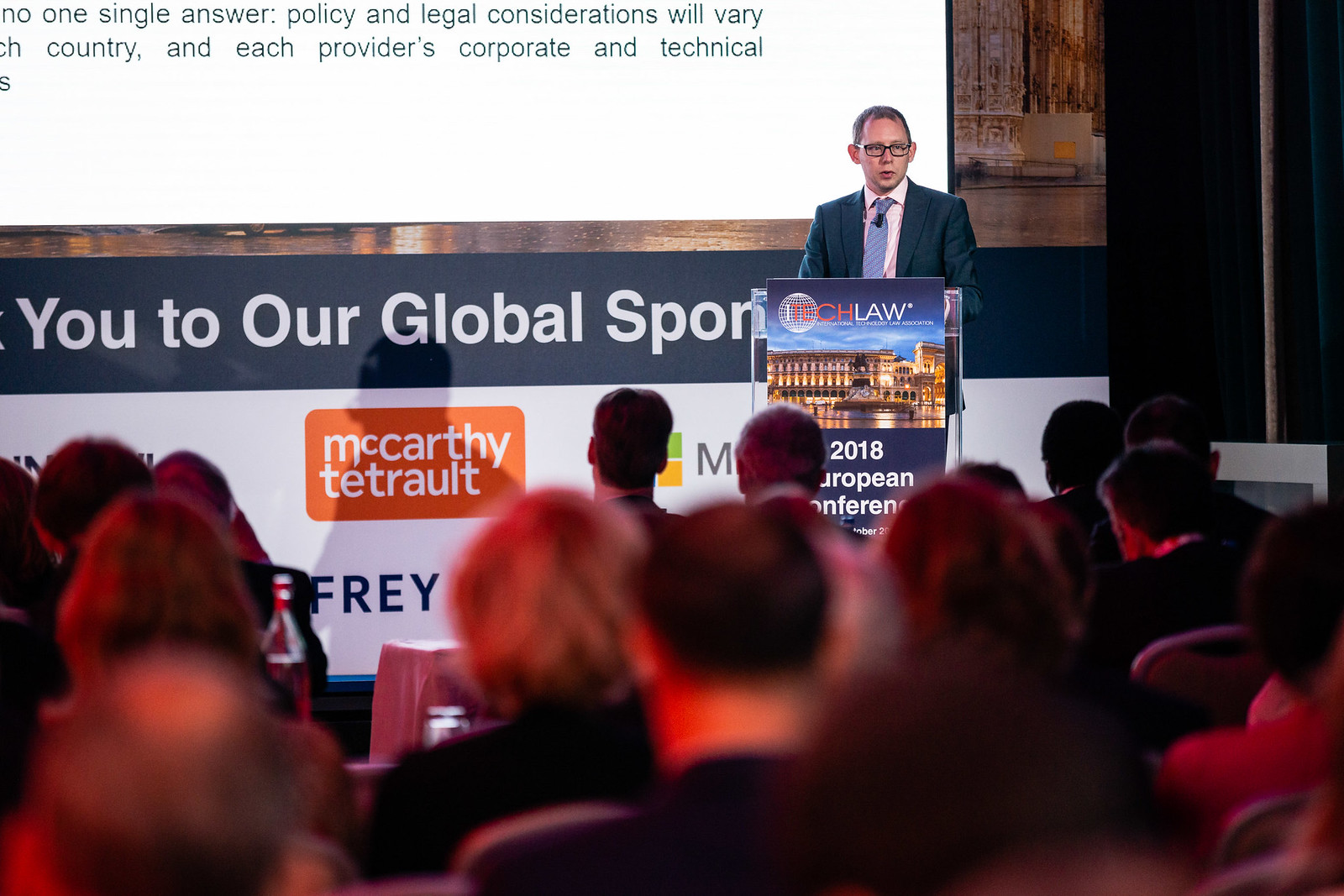The photograph captures an indoor conference event from a mid-crowd perspective, giving a clear view of the audience's heads as they attentively face the stage. The attendees, illuminated by a red light from behind, are seated and appear to be a mix of men and women, many of whom are dressed in suits. At the forefront, a man stands behind a clear podium emblazoned with "Tech Law" in red (or orange) and white letters. The podium also features an image of a night-lit building, suggesting architecture resembling the Roman Coliseum, and the inscription "2018 European Conference."

The speaker is wearing a navy blue suit complemented by a light blue tie and a salmon-colored shirt. He is also wearing glasses and appears relatively young, albeit with balding hair. Behind him, a large projection screen is visible, likely used for his presentation. Adjacent to the screen is a prominent banner partially obscured but readable enough to indicate a message of gratitude to the event's global sponsors, prominently mentioning "McCarthy Tetrault" in an orange box with white font. The photograph captures the essence of a formal, well-attended tech law conference, reflecting both the event's atmosphere and its detailed setting.